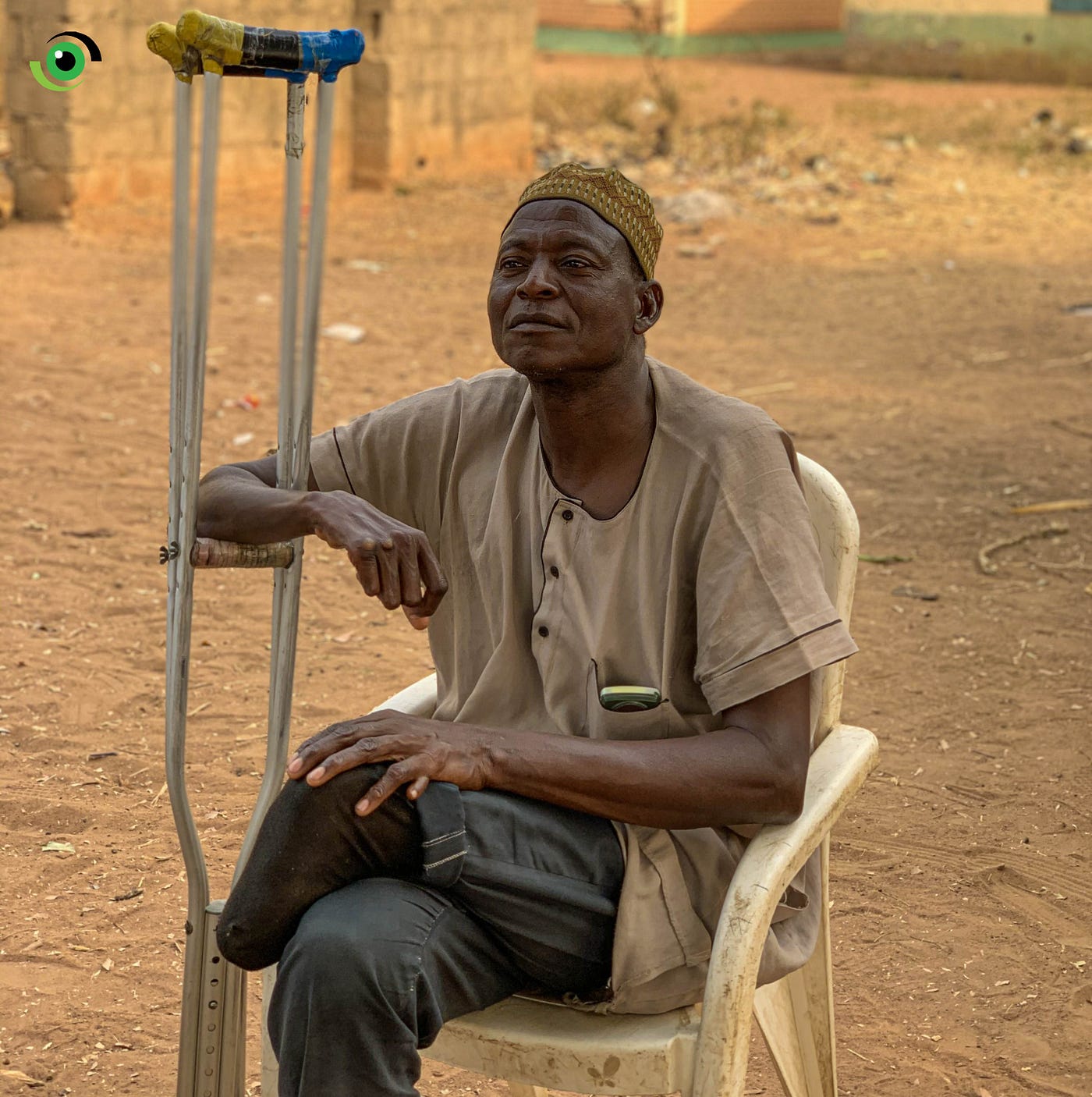The photograph captures a man of African descent, likely in his early to late 50s, seated in a small white chair on a dirt-covered ground. He is wearing a light brown short-sleeved shirt with something in the left front pocket and dark blue jeans. A small yellow knit cap adorns his head. His skin is dark, and he looks slightly towards the left. Notably, his left leg is amputated just below the knee, the remaining upper half resting over his fully extended right leg. He holds a crutch with his right hand, his elbow bent to support it. The crutch extends down and off the image at the bottom left and up to the left side of the photograph, featuring yellow, green, and blue accents at the top. In the background, there are portions of a stone wall and a house. At the top left corner of the image, there is a logo resembling an eye, composed of a green circle, a black swoosh, and a light green swoosh interspersed with black and white elements.